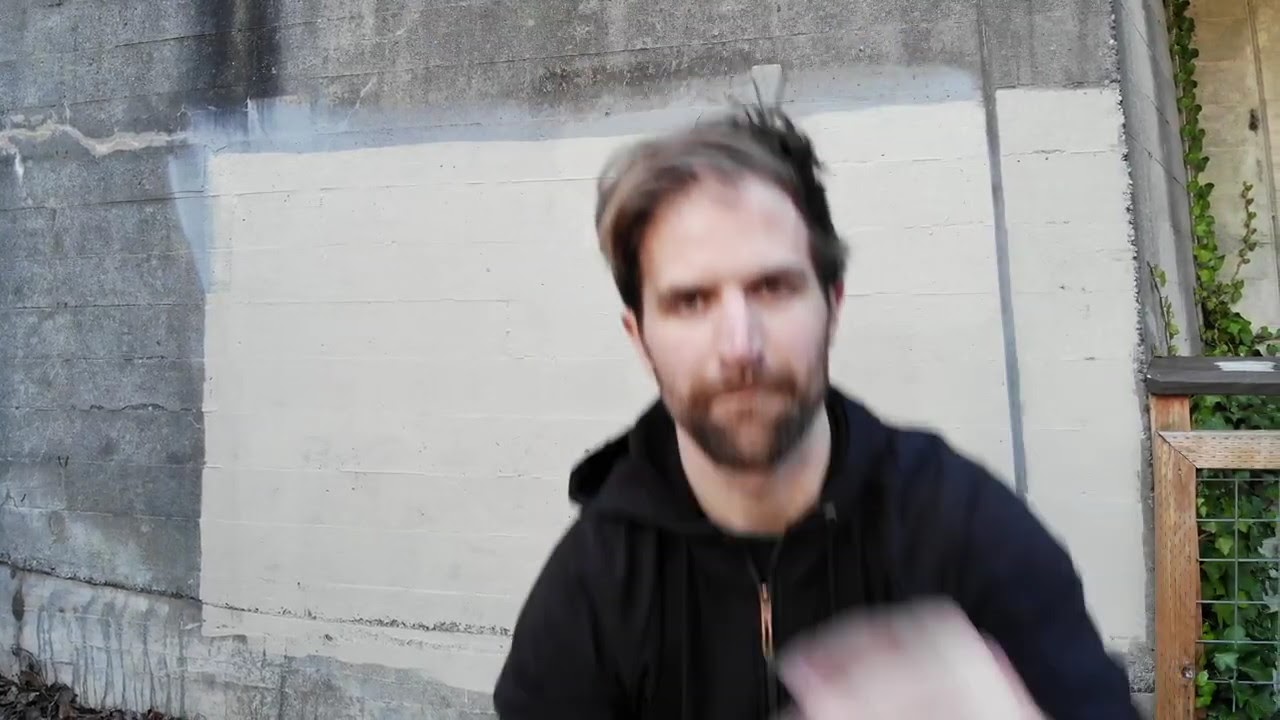This horizontal rectangular photograph, though a bit fuzzy, captures a white man with a receding hairline and black-brownish hair, sporting a black hooded sweatshirt. The man, who has a small beard and some stubble, is looking sternly ahead without a smile. There's noticeable motion blur suggesting he was moving when the picture was taken. In his hand, there's something indistinct and possibly shiny.

In the background, there's a concrete wall that's partially painted white, creating a square shape amidst the bare gray bricks. This gives the impression of an unfinished painting job. To the right side of the image, a gate can be seen with some bushes and vines peeking through. The photograph appears to capture both the man and the under-construction site he stands before, with the stark white section of the wall contrasting against the raw gray bricks and adding to the overall scene's dynamic feel.